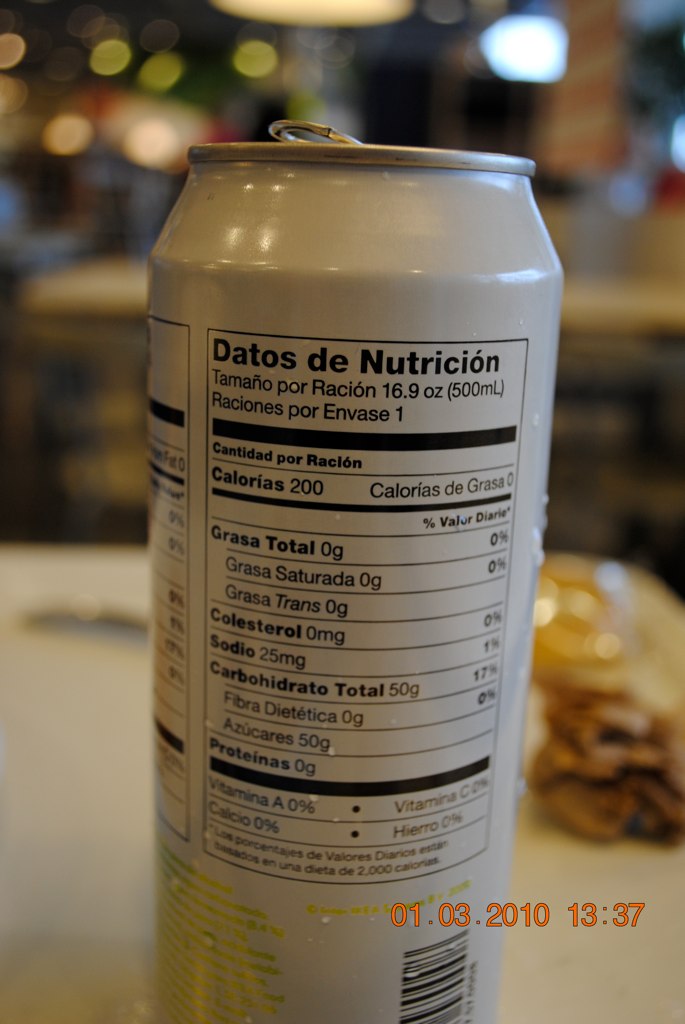This detailed side profile photograph captures the nutritional content label of a chilled, white drink can, printed in Spanish. The label details various nutritional facts, including 200 calories, cholesterol, sodium, carbohydrates, and vitamin content, with most vitamins listed as zero. The can, now sweating as if recently removed from a refrigerator, is set against a blurred background, making the can the focal point of the image. The photo was taken on January 3, 2010, at 1:37 PM, displayed in the 24-hour format as "13:37." The overall color scheme is neutral, with black lettering standing out clearly against the white can.